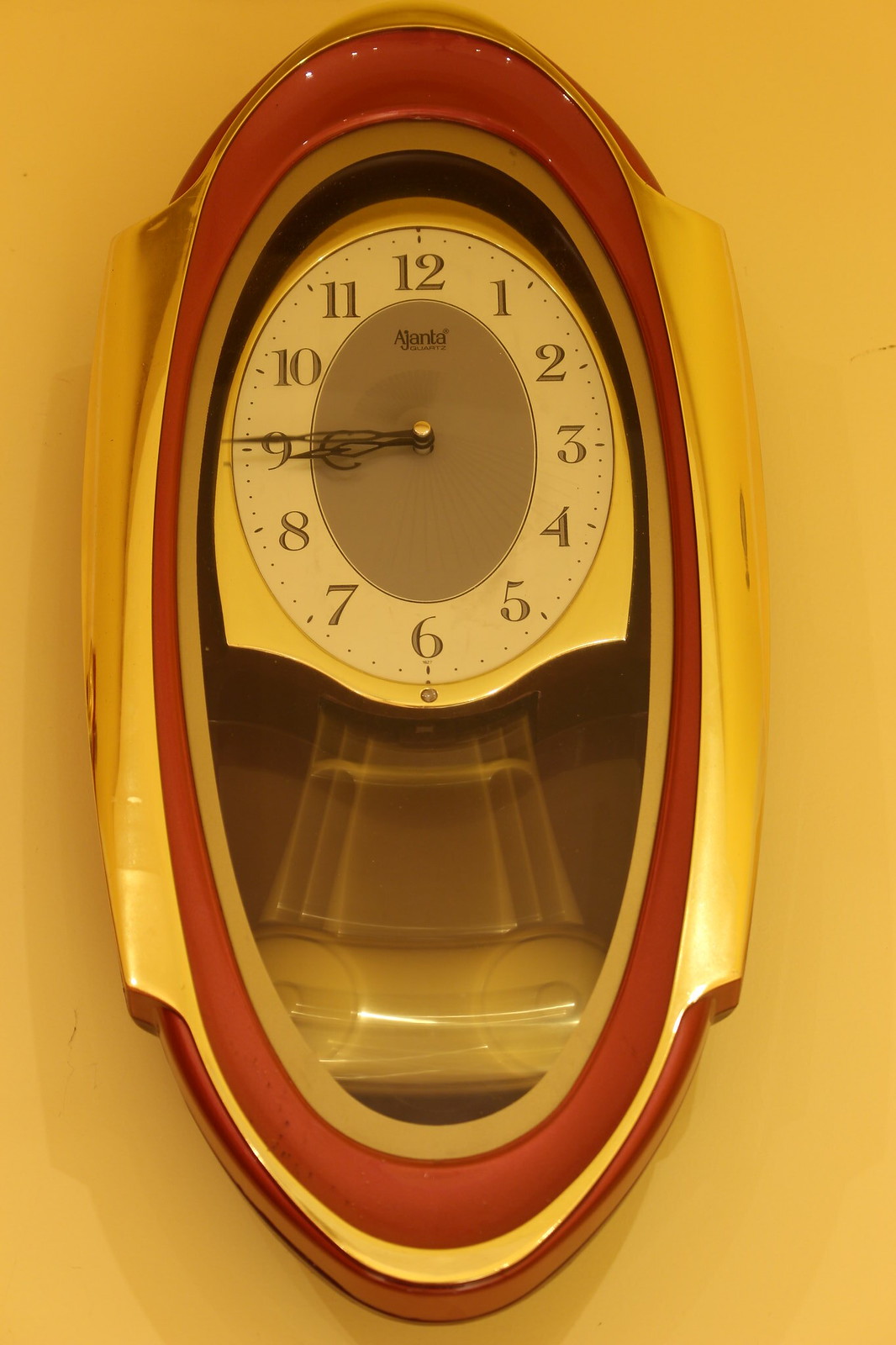This photograph captures an antique clock mounted on a beige wall. The clock features an oval shape, accented by a reddish-brown outer ring and an inner ring finished in a yellowish gold, both showing signs of wear and small chips, indicating its age. The clock face, also oval, clearly displays all 12 numbers, and is equipped with two hands showing the time as 8:46. Additionally, a visible pendulum swings underneath, its arc frozen mid-motion in this image, emphasizing the dynamic nature of the timepiece.